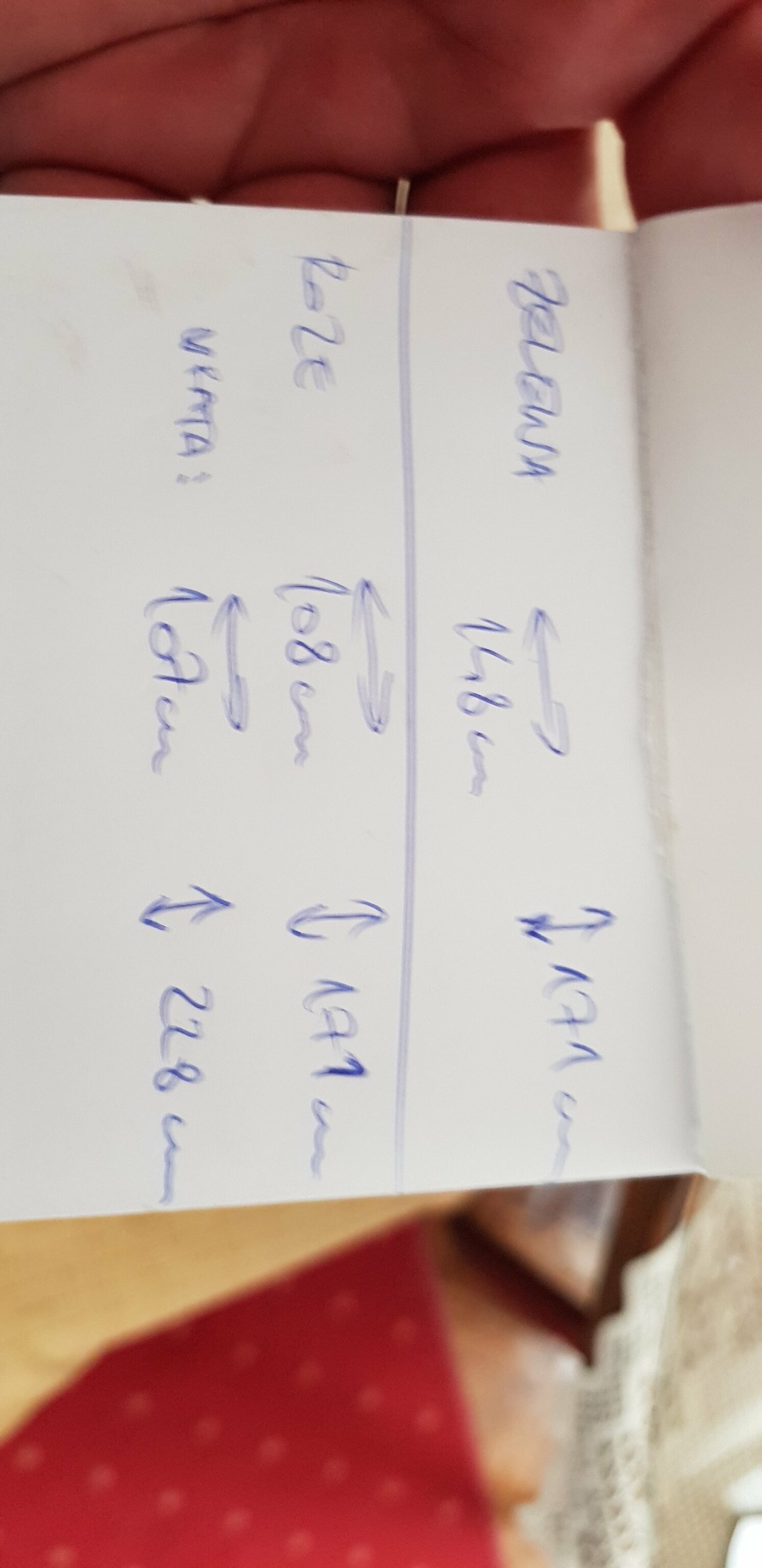The image depicts a close-up, blurry photograph of a rectangular notebook with blank white paper, held in someone's hand. The notebook is oriented sideways, and the focus is so tight that only one sheet of the paper is visible. Due to the poor focus, the writing on the paper appears indistinct. The top part of the paper seemingly reads "ZELEWA 148," accompanied by an arrow pointing in both directions. Below is another arrow pointing up and down, with "171 cm" written next to it. A line separates this section from the rest of the note. Following this, there are two more rows of text that appear to indicate measurements: "108 cm" with a bidirectional arrow, and "191 cm" with a vertical arrow. The last row is marked with "MRNTA" followed by "100 cm," "107 cm" with a horizontal arrow, and "228 cm" with a vertical arrow. The background of the photograph is indistinct, but a red object can be seen at the bottom, along with what seems to be a white tablecloth in the lower right corner.